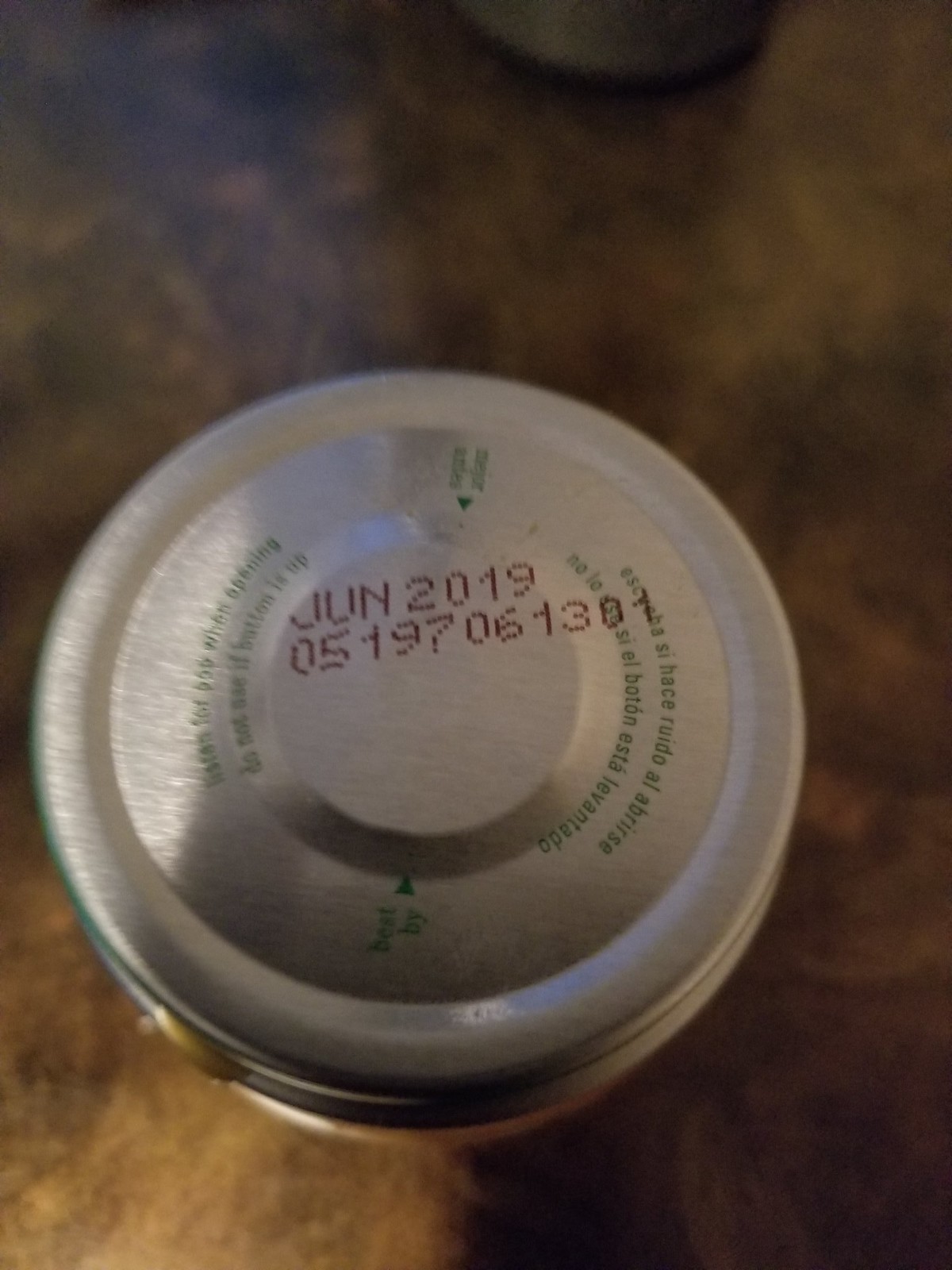This image captures a vertically aligned, slightly blurry photograph of a silver metallic lid, likely from a canister or jar, resting on a marble countertop that features a blend of black, brown, and cream colors. In the center of the lid, the bold, black text reads “June 2019” above a numerical code “05197061301.” Positioned towards the top edge of the lid is the phrase "Best By" accompanied by a small green arrow pointing towards the date. The lid also features text written in both English and Spanish in a circular formation around its center. Despite the blurriness, you can discern the typical indented bumps at the base, commonly seen on the bottoms of aluminum cans. The countertop, which appears to have a marbled pattern with hues resembling clouds of red and smoky grey, partially frames another indistinct object in the background.